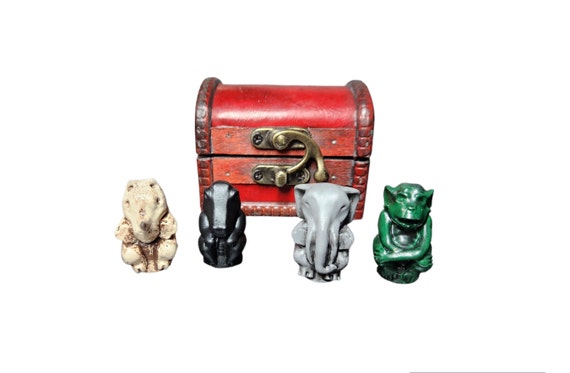This image showcases a group of intricately carved animal figurines arranged in front of a small, traditional red treasure chest with a worn golden latch. Set against a clean, white background, the scene highlights the detailed craftsmanship of each component. The treasure chest, with its characteristic curved top, appears to be made primarily of wood and measures approximately 12 to 14 inches in height. In front of the chest stand four figures, each around 3 to 4 inches tall, carved from materials resembling ivory or jade. From left to right, the figurines include a beige rhinoceros, a shiny black alligator-like creature, a gray elephant with a prominent trunk, and a green monkey. The monkey is notably crouched, with its arms wrapped around its knees, adding a unique touch to the collection. The arrangement and fine details suggest these are prized collector's items.